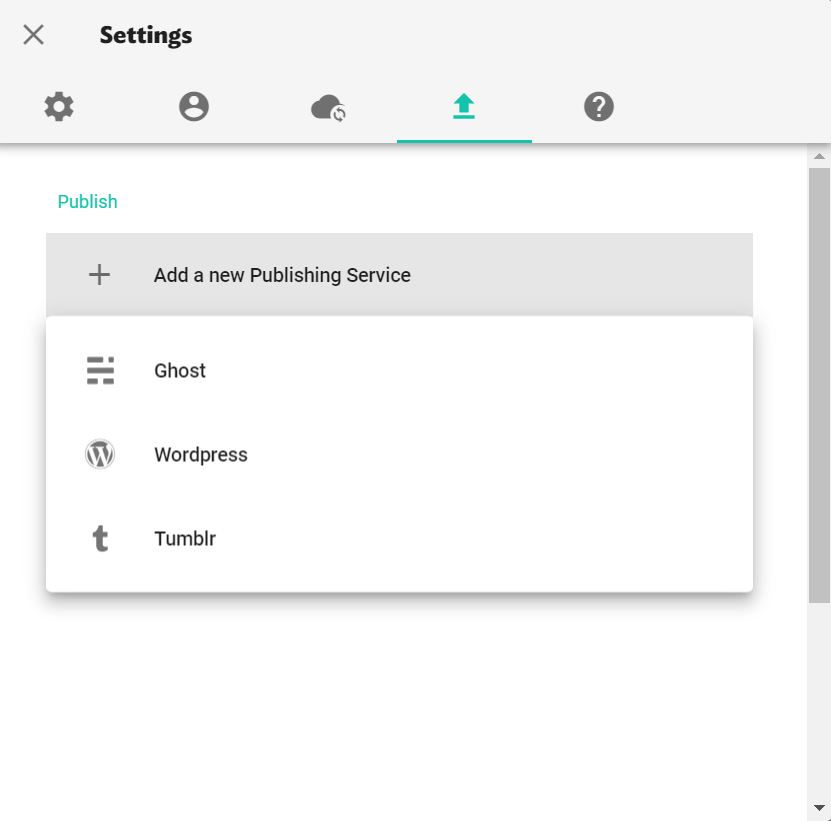This image displays the settings interface of a service, showcasing several options and icons at the top. Starting from the left, there's an "X" icon for closing the settings menu. Next to it, there are five neatly arranged icons in gray: a gear symbolizing settings, a person indicating login, a cloud for cloud services, an upward arrow for upload, and a question mark for help.

The currently selected option is "Publish," highlighted with a green upward arrow, signifying an active or selected state. The menu under "Publish" includes a section to "Add a new publishing service" and is followed by a scroll bar on the right side, indicating the presence of additional options or information off-screen.

Listed below the "Add a new publishing service" section are three publishing platforms: Ghost, WordPress, and Tumblr. Each option is presumably clickable or selectable for further configurations.

At the bottom of the section, the image has a white background with no further text or details, leaving it blank and uncluttered. This ample white space draws attention to the listed services and keeps the interface clean and straightforward.